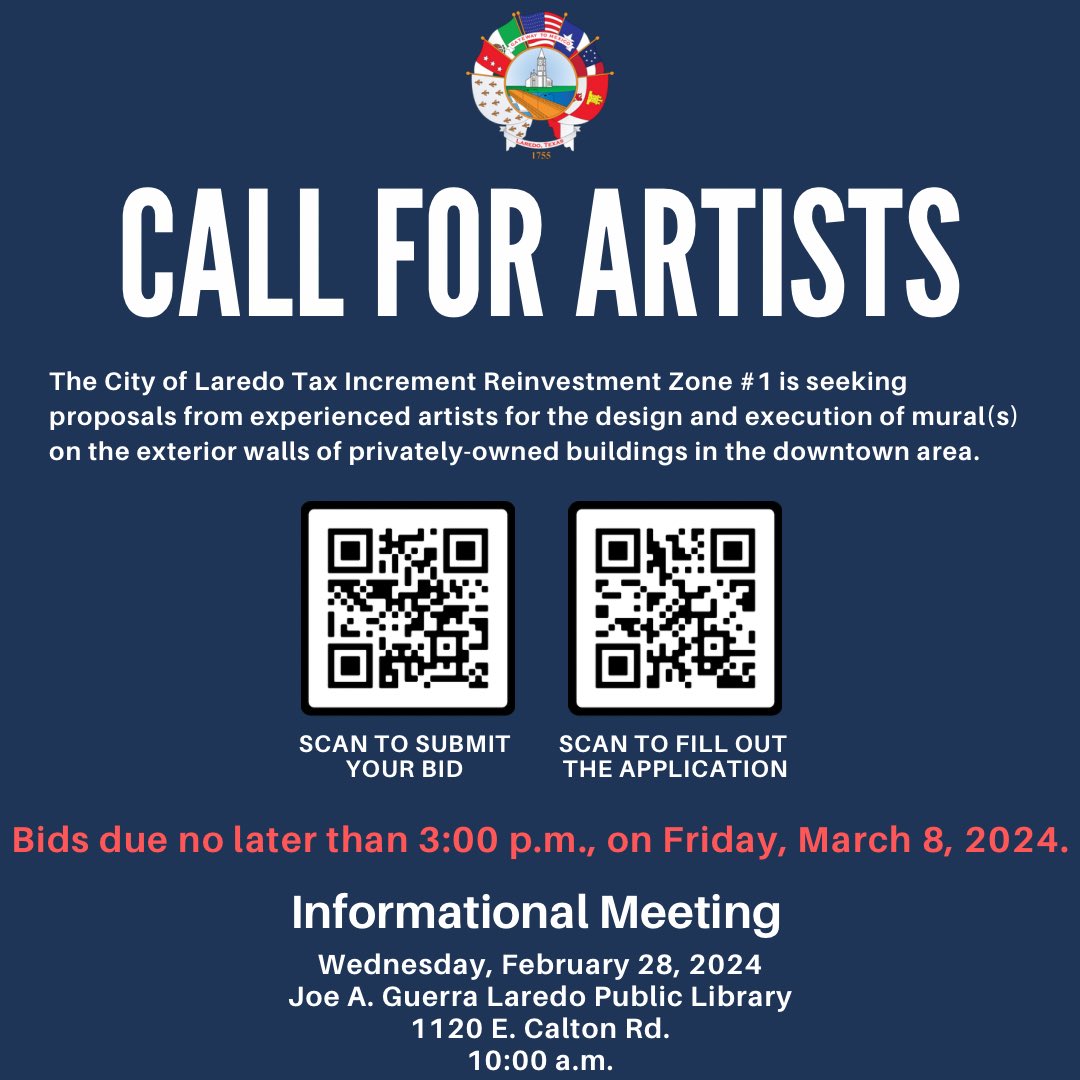The image is a square poster with a dark blue background. At the top, there is a round logo featuring colorful flags encircling a central building, possibly representing a lighthouse. Below the logo, in large all-capital white letters, is the text "Call for Artists." The next section in white text reads: "The City of Laredo Tax Increment Reinvestment Zone Number One is seeking proposals from experienced artists for the design and execution of murals on the exterior walls of privately owned buildings in the downtown area."

Underneath this announcement, there are two square QR codes. The one on the left has the caption "Scan to submit your bid," while the one on the right reads "Scan to fill out the application." Further down in red text, it states: "Bids due no later than 3 p.m. on Friday, March 8, 2024." Below this, in white text, is information about an informational meeting: "Wednesday, February 28, 2024, Joe A. Guerra Laredo Public Library, 1120 East Calton Road, 10 a.m."